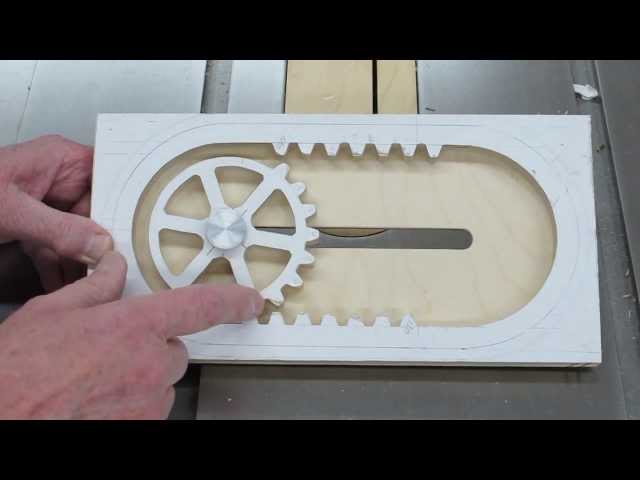In this screen capture from a video, an elderly man is demonstrating the mechanics of a white, rectangular wooden box with a unique inner mechanism. The box, roughly six inches tall and wide, features an oval cutout in the center where a round wheel with internal teeth resides. This wheel slides back and forth, catching on corresponding teeth located at the top and bottom of the box's interior. The interior background of the box is a light green wood, contrasting the painted white exterior. The man is pointing to one of the wheel's teeth, illustrating its function. This scene is set on a metal woodworking table, likely in a workshop under lighting that could be either natural or artificial. The focus is entirely on the box and the man's interaction with it, highlighting the intricate design and functionality of the wooden mechanism.